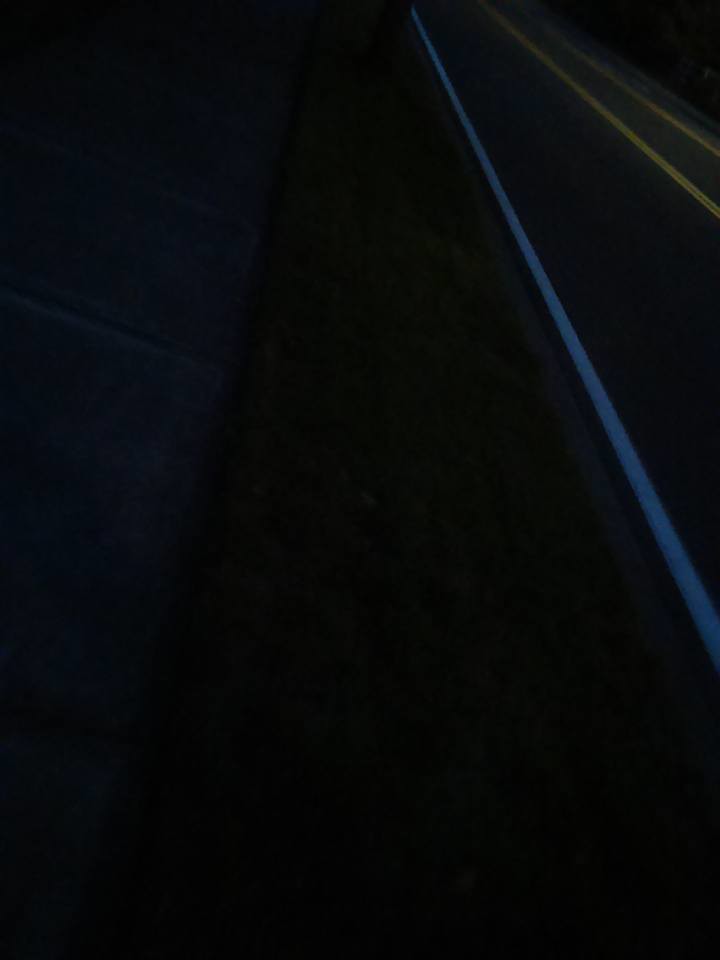The image is an outdoor nighttime photograph taken in very low light, with the camera pointed down toward the shoulder or grassy verge along the side of a road. In the upper right corner, there is a vertical white line marking the edge of a macadam road, alongside two diagonal or vertical double yellow lines, indicating it's likely a two-lane divided road. The bottom left portion of the photograph is entirely black, devoid of any discernible features. Additionally, there are no visible words, text, or print in the image. The faint visible elements suggest the image captures a small slice of a roadside scene, possibly an accidental snapshot.